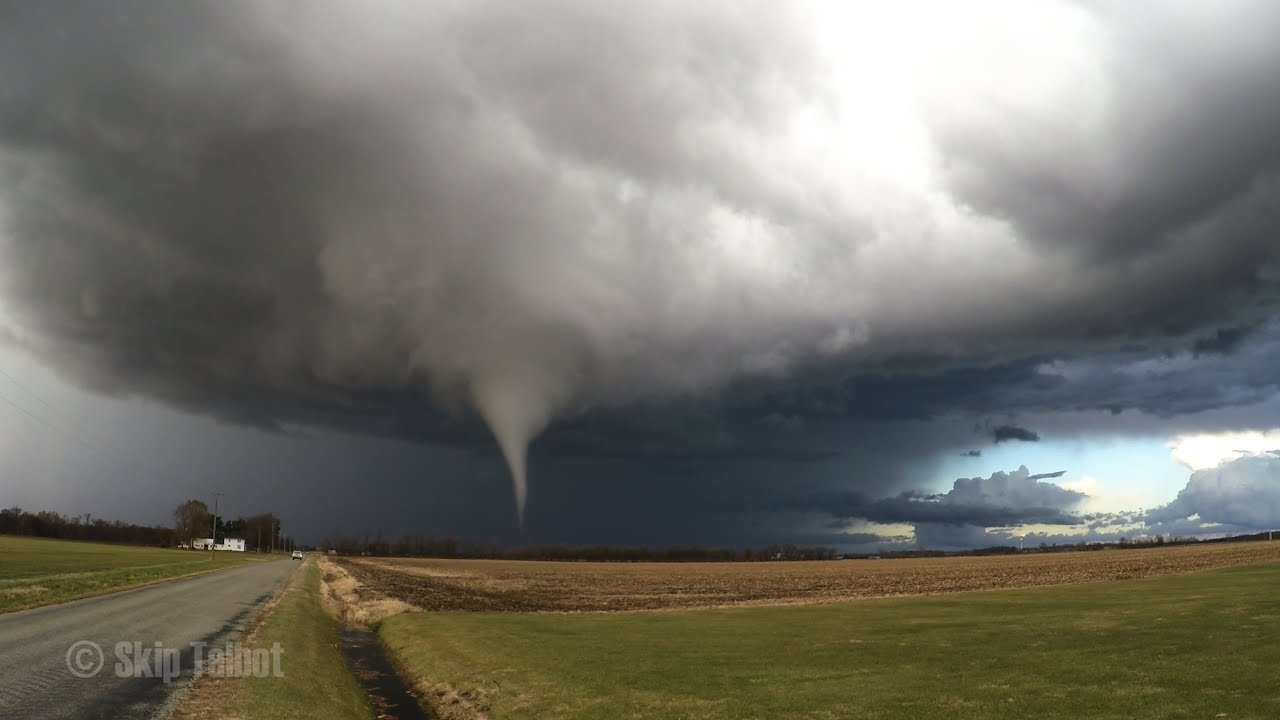In this dramatic panoramic photograph, we see a powerful tornado in progress set against a rural outdoor landscape. The tornado's funnel cloud, a light brown hue, stretches from the ground to a massive, angry-looking cloud above, consisting of swirling whites and dark grays. This cloud casts an ominous shadow over the landscape, with the funnel cloud appearing almost black where it touches the earth. Surrounding the tornado, the sky transitions from threatening browns and grays to a strikingly calm blue area on the right side, untouched by the storm. 

Below, the land is a mix of green grass and harvested brown soil. A gray gravel road cuts through the image from the bottom left towards the center, where a solitary car is seen driving towards the tornado. Off to the left side of the road, a white farmhouse and a line of trees stand on the distant horizon, dwarfed by the towering funnel and storm clouds. This rural scene captures the stark contrast between calm and chaos, with the serene blue sky on one side juxtaposed against the violent tornado and dark clouds on the other.